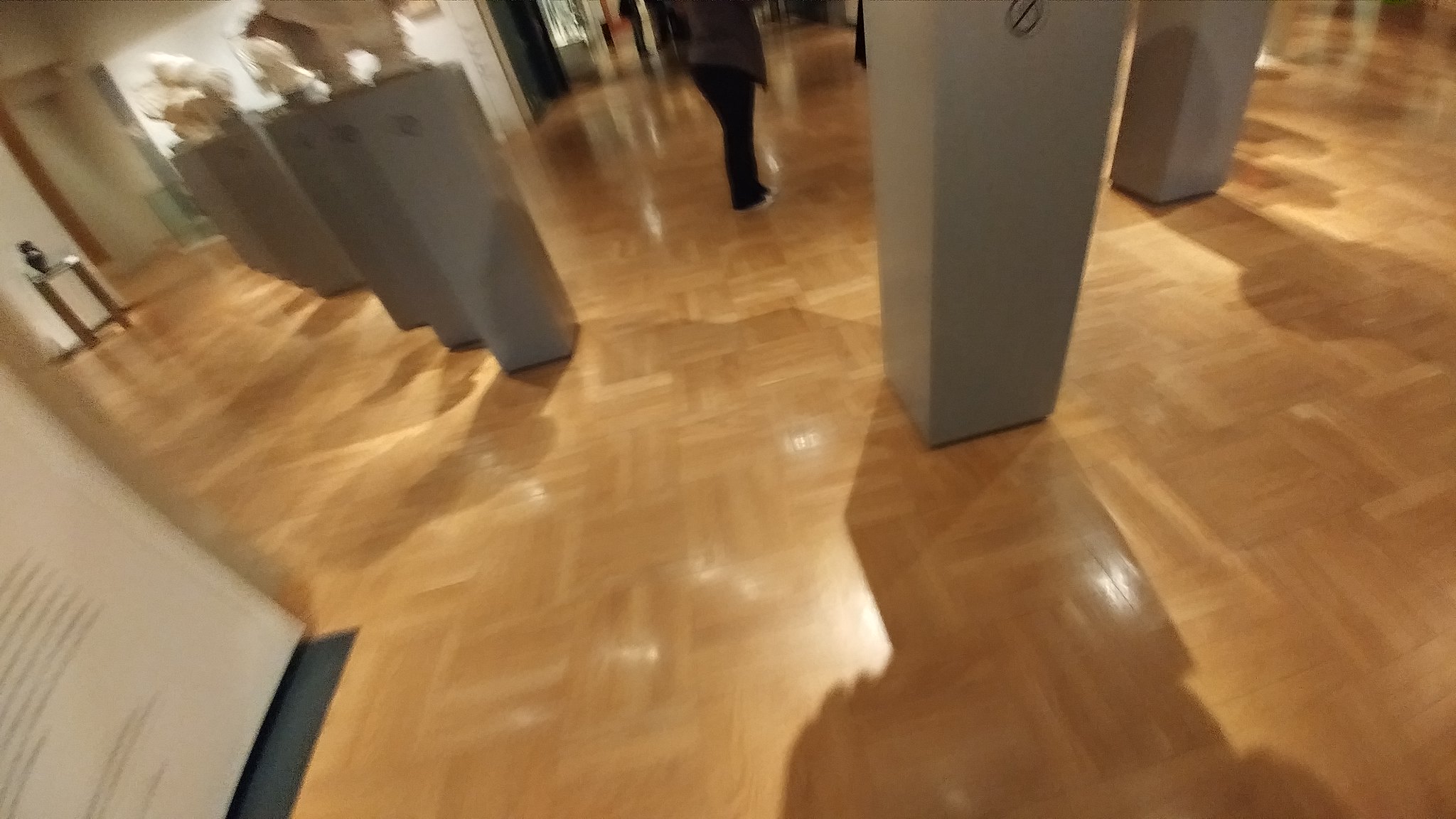The image captures the interior of what appears to be a museum or an art gallery, featuring a light wood-finished flooring that adds a warm ambiance to the space. At the center, a circular arrangement of gray pedestals draws attention, each subtly marked with a no-smoking symbol at the top. To the right, two of these pedestals are partially visible, hiding their displays. On the left side of the image, more pedestals come into full view, each showcasing a distinct sculpture, providing a glimpse into the curated artistic collection housed within the gallery.